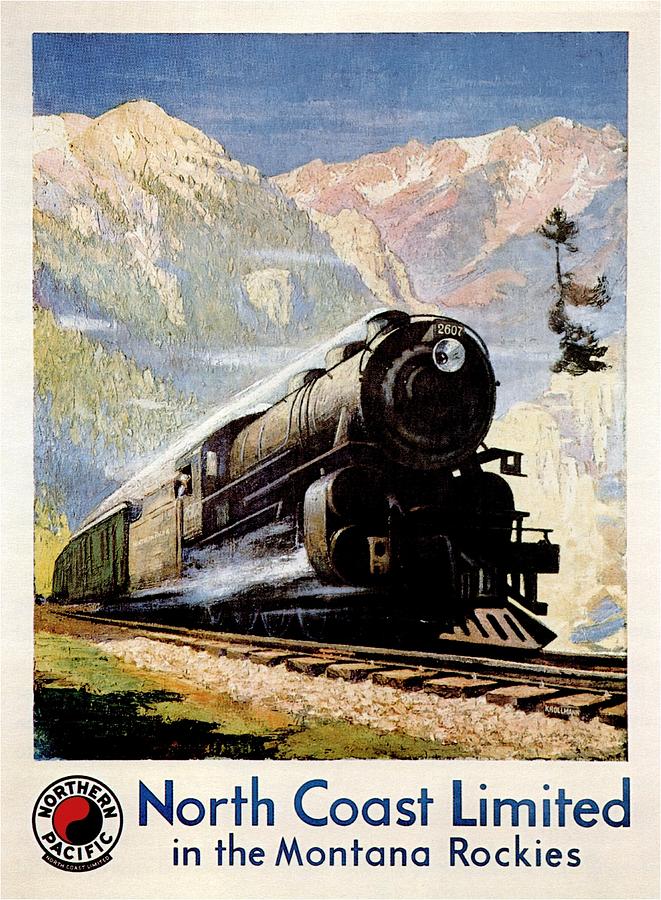The image is a refined reproduction or photograph of a vintage travel poster, rendered in a painterly style that suggests watercolor or acrylics. Central to the image is a large black locomotive, bearing the number 2607, speeding toward the viewer on brown and gray railroad tracks set against a backdrop of white gravel. The train is followed by a green passenger car. The captivating background features snow-capped mountain peaks with tree-covered flanks, bathed in sunlight, and giving way to bare summits, all awash in hues of pastel pink, green, and white. In the foreground, sparse ponderosa pine trees clinging to crags and green grass are visible, casting shadows that further add to the depth of the scene. The sky is a serene blue, enhancing the vibrant play of colors throughout the image.

At the bottom of the poster, in blue font, it reads "North Coast Limited in the Montana Rockies, Northern Pacific," accompanied by the Northern Pacific logo—a yin-yang-inspired design featuring nested red and black paisley shapes—positioned in the bottom left corner. The upper right corner of the poster includes an additional detail, a small illustration resembling a bonsai tree. The overall effect is a visually rich and nostalgic homage to the romance of railway travel through the majestic Montana Rockies.